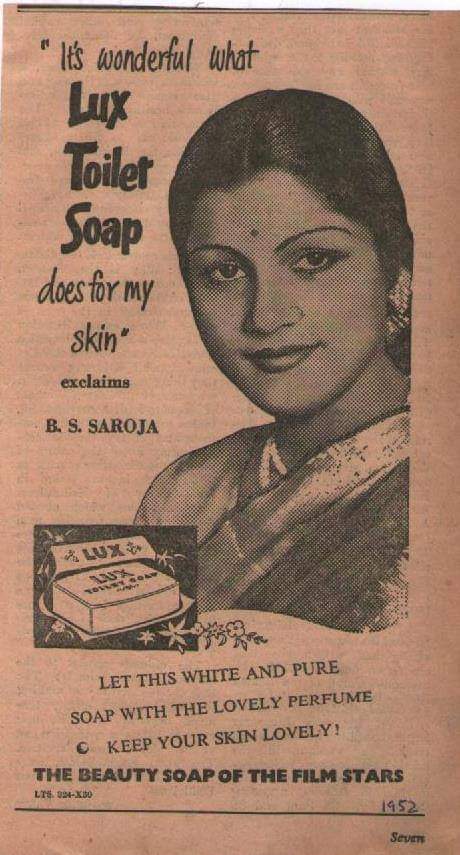This is a narrow, vertically aligned rectangular vintage advertisement, resembling a newspaper clipping from 1952. The background has an aged, brownish hue. At the top left, there is a quote in bold black letters stating, "It's wonderful what Lux toilet soap does for my skin." Featured prominently to the right of the text is a large image of a young Indian woman with dark hair pulled back, thin and curved eyebrows, and a dot in the middle of her forehead. She is smiling directly at the viewer, and appears to be wearing a sari or robe with a beaded necklace. Below her image, there’s an illustrated bar of Lux soap inside a square. The text beneath the soap illustration reads, "Let this white and pure soap with the lovely perfume keep your skin lovely." Centered at the bottom of the ad, it says, "The beauty soap of the film stars." In the lower right corner, the year "1952" is handwritten, along with the word "seven" printed just below it, possibly indicating a page number.